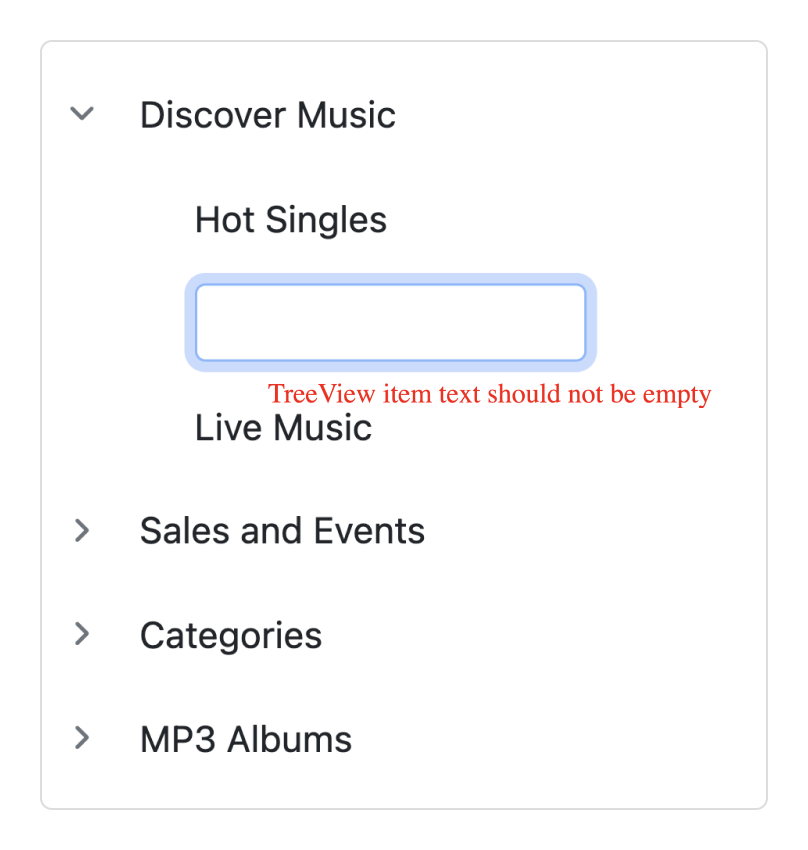A vertical screenshot of a digital interface, likely from a computer or smartphone device, displayed on a white background. At the top of the screen, "Discover Music" is prominently featured in black text, accompanied by a small down arrow. Directly below this, the heading "Hot Singles" is displayed. 

Beneath "Hot Singles," there is a white box outlined in blue, which is currently empty. Following this, a red error message states, "Tree View Item Text should not be empty." 

The interface continues with the label "Live Music" in black text. Further down, an arrow points to the right, directing attention to the category labeled "Sales and Events." Another right-pointing arrow follows, linked to the "Categories" section.

At the bottom of the screen, a final right-pointing arrow directs to the "MP3 Albums" category, also in black text.